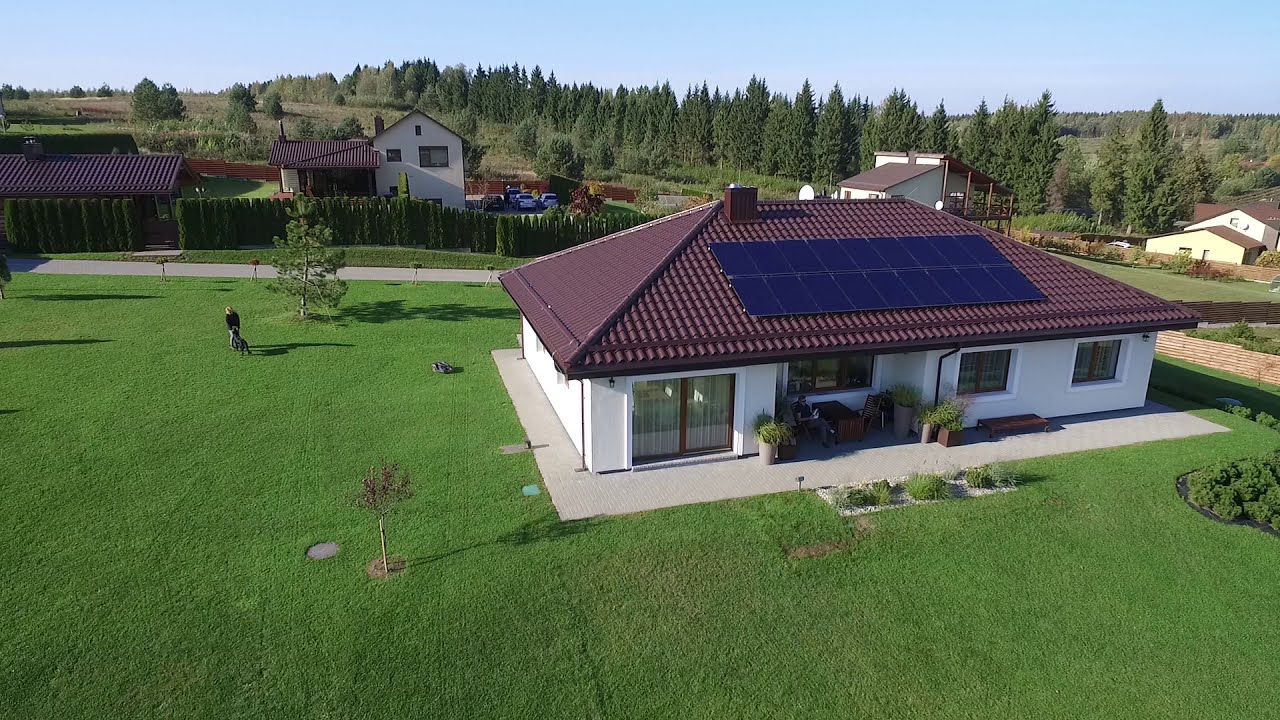The drone-shot image showcases a primarily white, newly built house positioned slightly to the right of the center in a lush suburban or rural area. The house features a brownish-red tile roof with a Japanese stylistic influence and is adorned with solar panels and a chimney at its peak. The ground level includes a green front door and sliding patio doors on the left side. Surrounding the house is a large, vibrant lime-green lawn with scattered plants, bushes, and small trees. To the rear of the property, across a road, stand several other white houses, all featuring similarly styled dark maroon roofs with tall hedges serving as fences. The background features an array of green-leaved trees set against a light blue sky, indicating a recent development with a natural incline suggesting nearby hills.